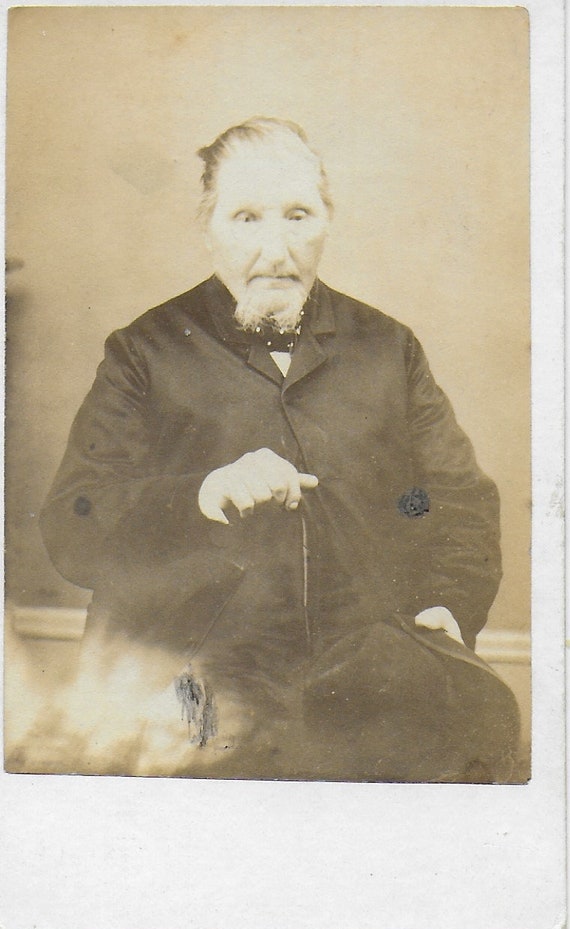The image is a very old sepia-toned photograph that likely dates back to the 18th or early 19th century. It depicts an older, light-skinned man with a dark receding hairline and a white goatee, wearing a black collared jacket buttoned at the front and a black bow tie with white polka dots. His white shirt is visible beneath the coat's collar. He is seated and holding a cane in front of him, his hands positioned centrally. There is an unusual six-fingered right hand clearly visible, suggesting the image might be AI-generated. The man appears to be looking slightly downward, giving him a distant expression. The top of the photograph is filled with a light sepia tone, while the bottom left corner shows signs of yellow glare and fading. There are also two black marks: one near his right elbow and another before his left elbow. The photograph has a slightly grainy texture, contributing to its aged appearance.